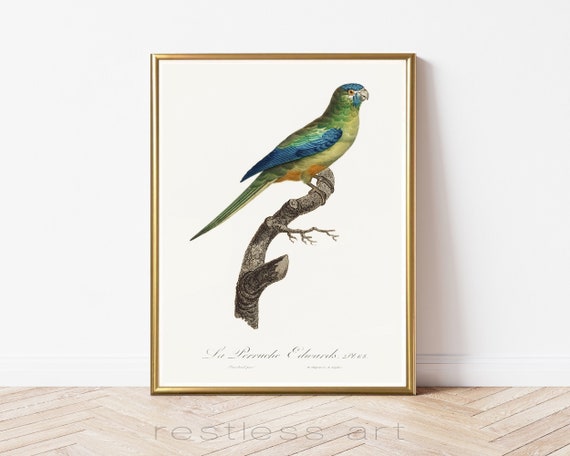This image features a framed hand-drawn poster of a parrot leaning against a white wall. The frame is gold, and the poster showcases a parrot perched on a craggy, leafless tree branch. The parrot is depicted in a side profile, facing right, with green on its belly, tail feathers, and back, and blue on its head and outer wings. A touch of orange is visible on the lower belly, and the parrot's beak is gray. The artwork rests on a light-colored wood floor arranged in a herringbone pattern. The background of the poster is beige, and there is light, cursive French text along the bottom that is difficult to read. A watermark saying "restless art" spans the bottom of the image in gray.